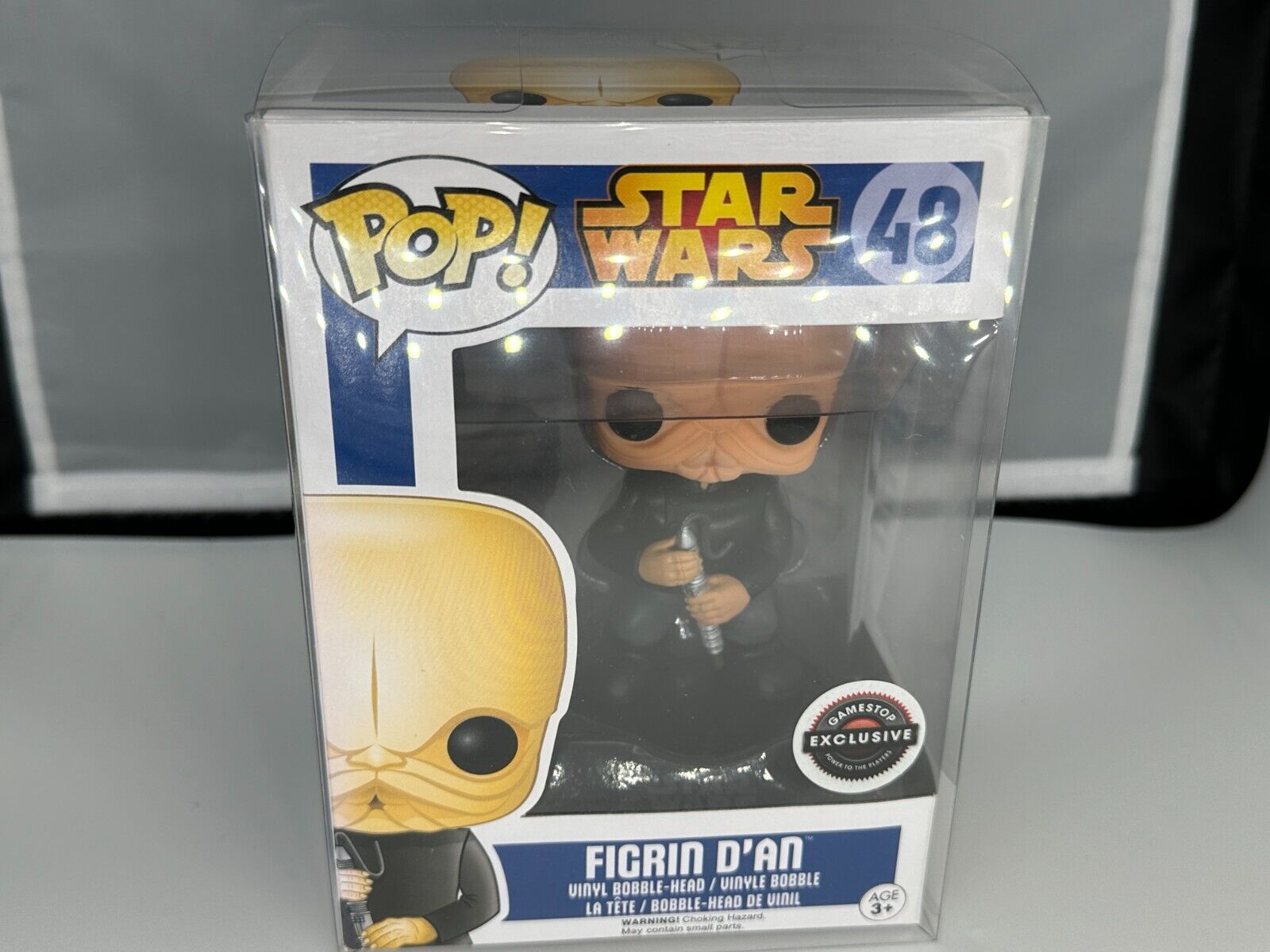This is a photograph of a Funko Pop vinyl bobblehead figure from the Star Wars franchise, specifically depicting the character Figrin D'an, known for his appearance in the Mos Eisley Cantina band. The figure is still in its box, which features a clear plastic window in the center that allows a view of the character. Figrin D'an is illustrated with a flesh-colored face, large black eyes, and numerous wrinkles, giving him an alien appearance. He is holding what appears to be a musical instrument associated with his character in Star Wars.

The box itself has a distinct comic-book style design with the following details:
- In the top left corner, the word "Pop!" is displayed in bold yellow letters with a lighter gradient toward the bottom, accompanied by an exclamation point.
- The Star Wars logo is prominently featured in the middle of the top section.
- The number "48" is indicated to the right of the logo.
- There's a circular black sticker on the right side of the box stating "GameStop Exclusive."
- At the bottom of the box, the name "Figrin D'an" is written in white letters within a blue rectangle.

On the lower left corner of the box, an illustration of the character displays his wrinkled head and large black eyes, matched with a black outfit. Additional details such as "Vinyl Bobble-Head" are mentioned, accompanied by various language translations and a "3+" age warning symbol seen on the bottom right. The backdrop of the photo includes a white table and a gray wall or bag with white trim, giving the scene a simple, non-stylized appearance akin to what a collector might use for an online listing.